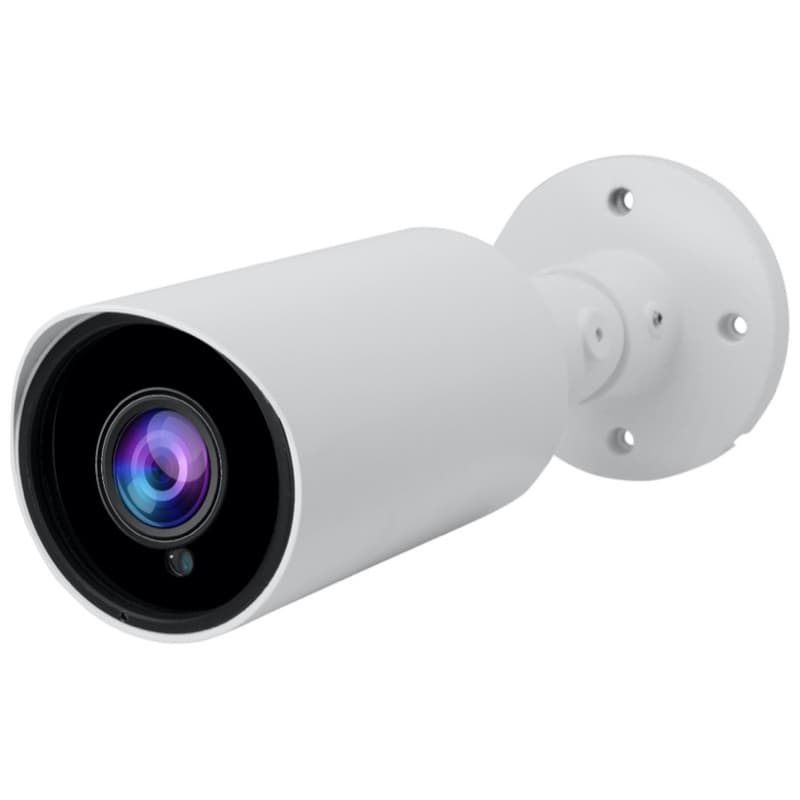This detailed close-up photograph features a security camera against a white background, laying horizontally on its side. To the right of the image is a round mounting base equipped with three to four evenly spaced drill holes, designed for secure wall attachment. Extending from this base is the camera's conical white plastic body that narrows before widening at the lens. The left side of the image prominently displays the black mechanical part of the camera lens. The lens itself, situated at the center, exhibits an iridescent reflection of vibrant purple and blue shades, adding a striking visual element. Below and near the base, there is an additional, smaller hole, highlighting the clean, sharp, and mechanical design of the camera.